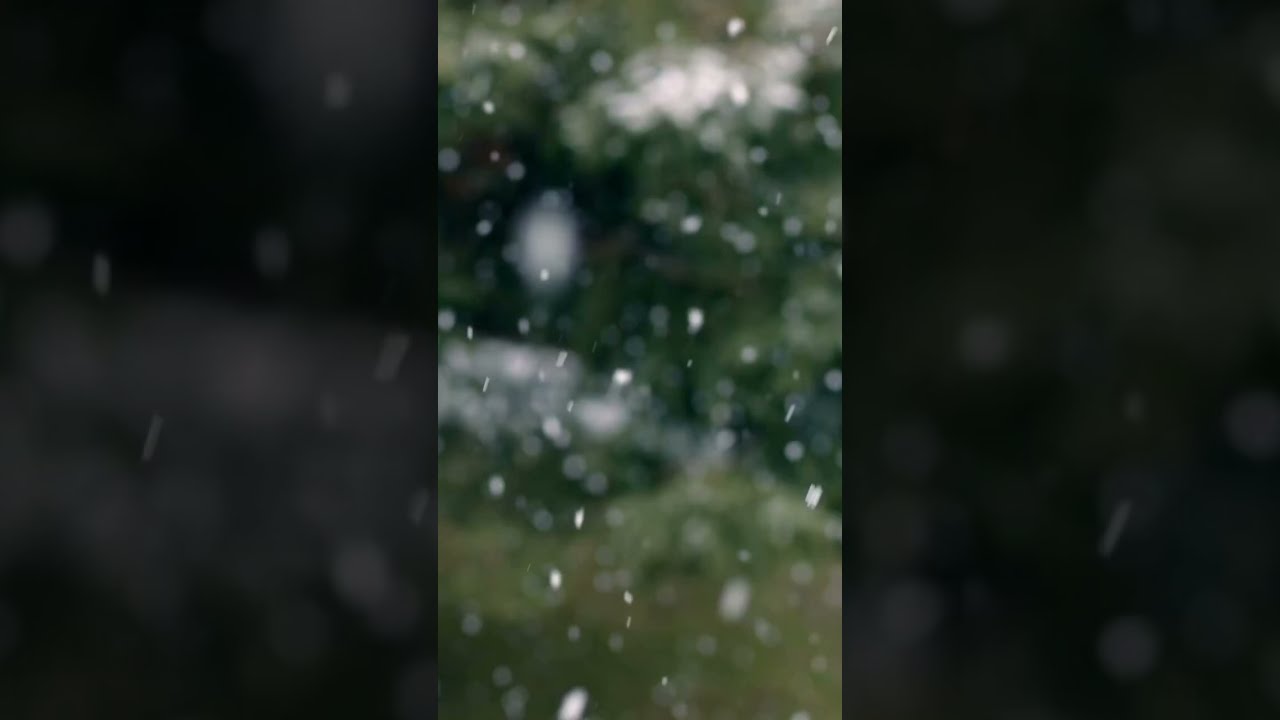The graphic is a horizontally-oriented rectangular image divided into three vertical panels. The central panel, which captures most of our attention, features a highly blurry photograph of an outdoor scene. It looks like a view through a window, displaying green bushes or grass with white patches potentially indicating falling snow or rain droplets. These blurs add to the difficulty of interpreting the exact scene. The left and right panels contain close-up sections of this central image, but are overlaid with dark or black layers which obscure the details, emphasizing the central panel. The left panel has a gray background with visible watermarks, while the right panel displays a dark green background also marked by water spots.